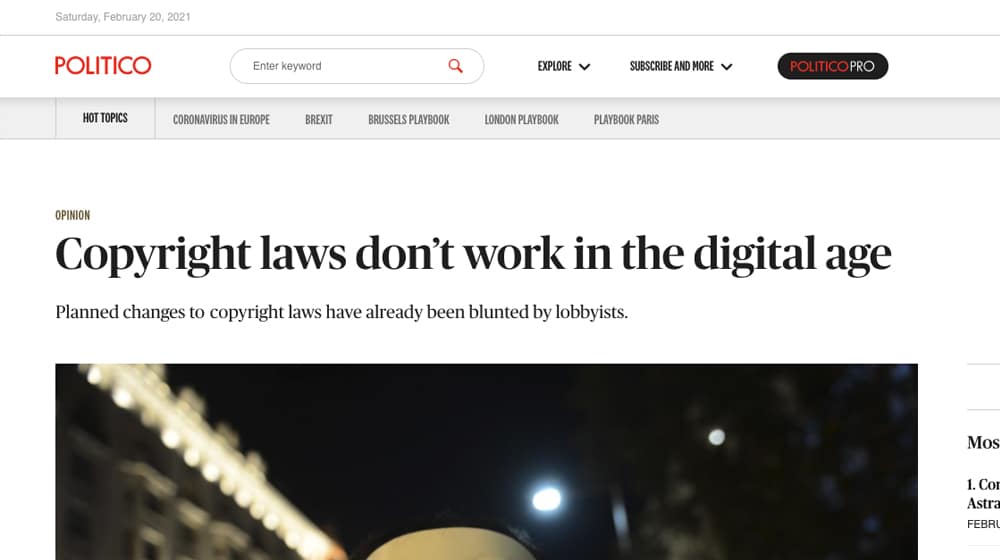This is a screenshot captured from the website Politico dated Saturday, February 20th, 2021. The date is displayed in a small, light gray font in the upper left-hand corner of the screen. Beneath the date is a gray separator bar. Directly below the separator, the website’s name "POLITICO" is prominently displayed in all capital letters and an orange font. Adjacent to the website’s name, towards the right, is a search bar, followed by the "Explore" option accompanied by a drop-down arrow. Next to "Explore," there are options labeled "Subscribe" and "More," each with their own drop-down arrows. Further to the right, there is a black button labeled "POLITICO PRO."

A portion of an article begins just below these navigation elements, showing the visible title "Copyright Laws Don't Work in the Digital Age," although part of the article is cut off due to the manner in which the screenshot was taken.